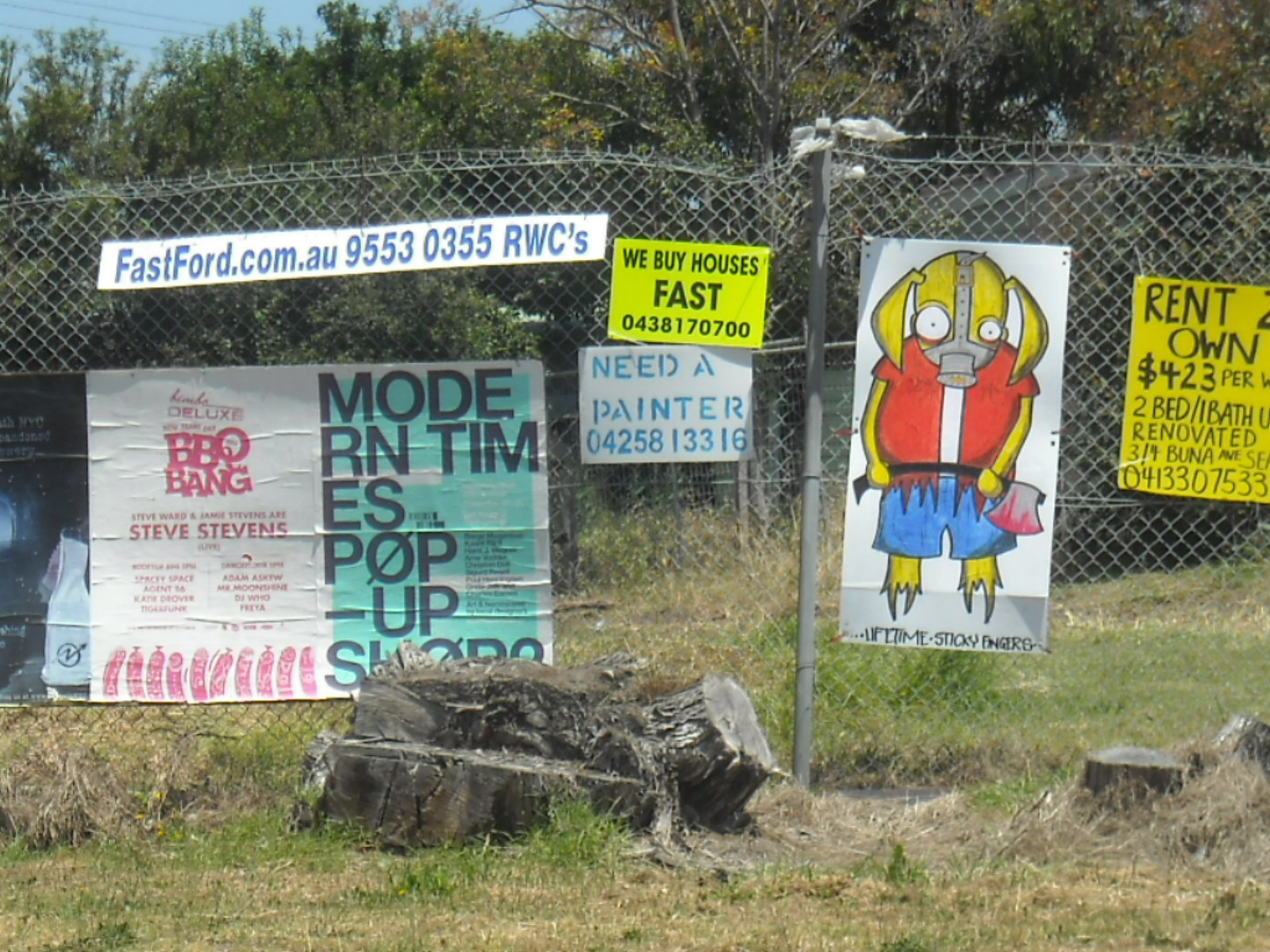The image, taken outdoors in a run-down area, features an old, rotting tree stump surrounded by overgrown green and yellowish grass in front of a weathered chain-link fence. The fence is adorned with multiple signs, including a prominent yellow "Rent to Own" sign that partially reads "423 Per ..." and mentions "2 bedroom, 2 bath" and "renovated." Nearby, another yellow sign declares "We Buy Houses Fast," and below it, a white sign offers "Need a Painter?" with a contact number. On the left, a white sign reads "Bassboard.com.AU95530355RWCs," and below it, another white sign advertises "BBQ Bang Steve Stevens." On the right side, amidst the clutter of advertisements, a striking cartoon graphic depicts a yellow figure in a red shirt and blue shorts, ominously holding a bloody hatchet and wearing a gas mask. In the background, there are trees in varying stages of shedding their leaves and a patch of blue sky visible in the top left corner.